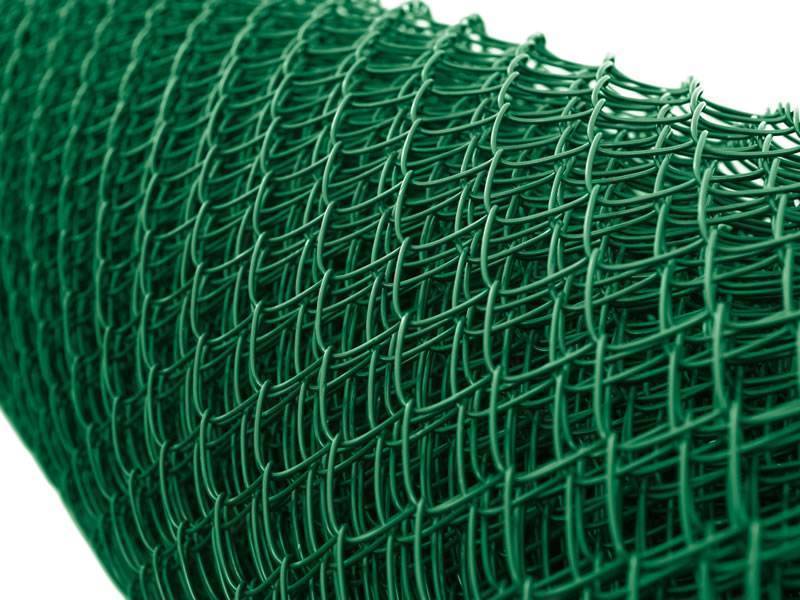The photograph showcases a close-up view of a large, green, tightly wound net or chain link fencing, coiled in a cylindrical roll. Positioned diagonally from the top left to the bottom right corner against a stark white background, the netting is detailed with tightly interconnected loops resembling arches or hooks, creating a dense pattern. A subtle glow accentuates the texture of the netting from the top right, while a bokeh effect blurs the edges, particularly towards the left side. This side shot, likely intended for product detailing, reveals the substantial layers and intricate design of the green-coated material, often used for fencing, making it suitable for display on platforms like Home Depot or similar retailers.